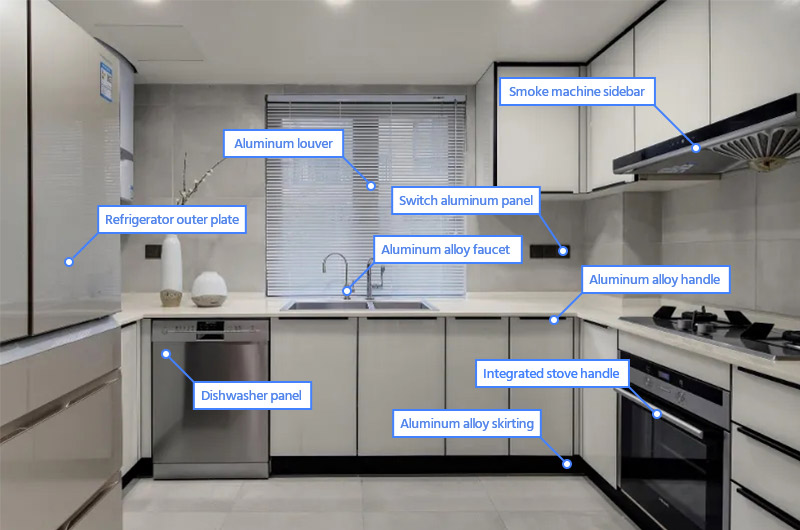The image depicts a modern, sleek, and predominantly white kitchen with stainless steel and silver-colored appliances. The kitchen features white tile floors, white cabinets on the right side, and a white ceiling. Central to the layout is a double sink situated in front of a window adorned with white blinds. Above the dishwasher on the left side of the sink are a couple of white vases.

Elements within the kitchen are meticulously labeled with blue text on white rectangular labels, each pointing out specific features with blue lines ending in white dots. Notable labels include "refrigerator outer plate," "dishwasher panel," "integrated stove handle," "smoke machine sidebar," "aluminum louver" (located behind the sink at the window), "aluminum alloy faucet," "aluminum alloy skirting," and "switch aluminum panel." The kitchen exudes a minimalist and somewhat barren aesthetic, suggesting that it serves as a showroom or display space rather than a functioning household kitchen. All labeled parts highlight the detailed materials and components, emphasizing the extensive use of aluminum alloys in the design.